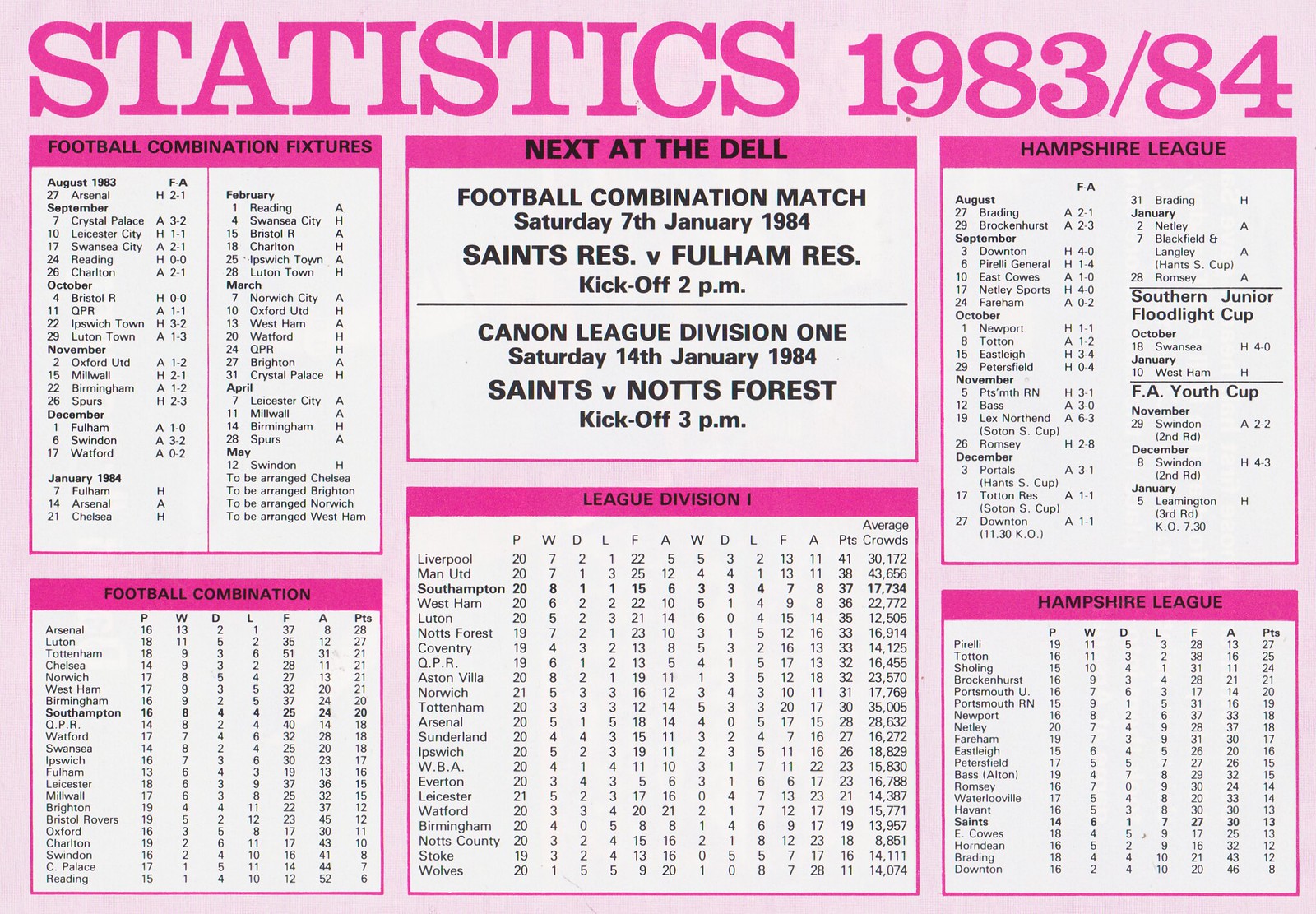The image is a large, horizontal rectangular graphic resembling a spread from a game program, predominantly themed in pink. At the very top, in bold dark pink serif font, the text "STATISTICS 1983/84" spans the width of the graphic. Below this headline, the layout is divided into six panels, each framed in darker pink with a corresponding pink banner at the top, containing titles in black letters.

On the top row, the first panel on the left is titled "Football Combination Fixtures" and features two columns with names and statistics. The top center panel, labeled "Next at the Dell," contains detailed event information in black letters against a white background: "Football Combination Match, Saturday, 7th January 1984, Saints Res. vs. Fulham Res., Kickoff 2 p.m." A black horizontal line separates the next section, "Cannon League Division 1, Saturday, 14th January 1984, Saints vs. Notts Forest, Kickoff 3 p.m." The top right panel is dedicated to the "Hampshire League," displaying columns of names and statistics.

The bottom row mirrors the top in structure, with the first panel titled "Football Combination," containing several columns of numerical statistics. The center panel, slightly wider, is labeled "League Division 1" and lists team names alongside various performance metrics in multiple columns. The final panel on the bottom right is another "Hampshire League" table, again filled with names and statistical data. The entire spread is visually unified by its light pink background and consistent use of darker pink elements.